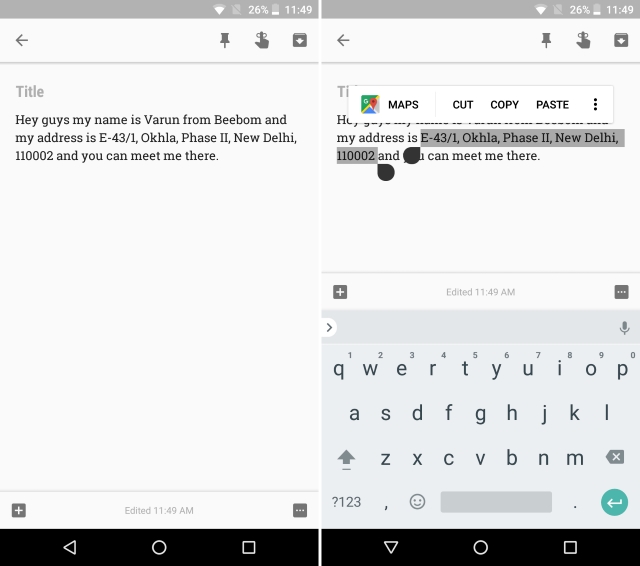In the provided screenshots captured on a mobile device at 11:49 a.m., the battery level is shown to be at 26% and Wi-Fi is enabled. 

The first screenshot features a user interface with several buttons at the top, including an arrow pointing left, a pin, an icon of a hand with a string around a finger, and a download button. The background is predominantly white with black text, while the title, written in gray, states: "Hey guys, my name is Varun from BeeBomb, and my address is E-43-1, Okhla Phase 2, New Delhi, 110002. You can meet me there." The information was edited at 11:49 a.m.

The second screenshot shows a highlighted segment of Varun's address with contextual options like "Maps," "Cut," "Copy," and "Paste" available in a contextual menu. The background of the highlighted text is gray. The QWERTY keyboard is visible at the bottom of the screen, indicating text entry or editing. The timestamp for the edit in this screenshot is also 11:49 a.m.